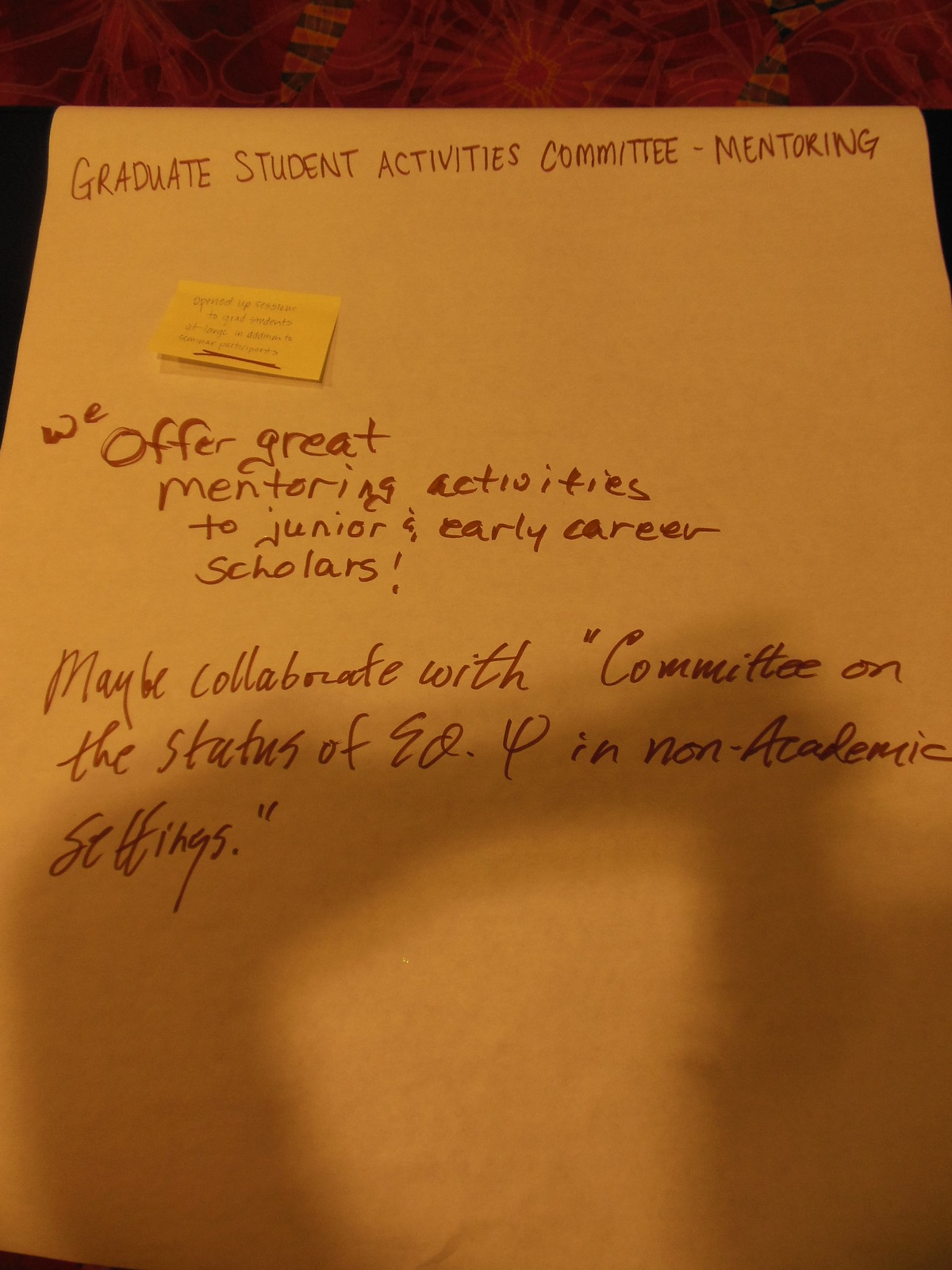The image depicts a piece of paper, possibly the back of a manila envelope, placed on a mahogany table. The paper has a yellow sticky note attached to its top left corner, which is difficult to read and might even be upside down. The entire scene is bathed in a tan filter with sunlight or regular indoor lighting casting shadows and highlights, including a prominent triangular splotch of light pointing downwards at the bottom right.

The paper contains a handwritten note in black ink, which reads: "Graduate Student Activities Committee - Mentoring." Further down, the text continues with: "We offer great mentoring activities to junior and early career scholars!" The message is centered left and skips a line before transitioning into a more cursive style, stating: "Collaborate with 'the statutes of EOP' in non-academic settings." Some areas of the text are obscured by shadows, rendering parts of it illegible.

In the background, a bit of carpet and more of the mahogany table are visible, suggesting a cozy, indoor environment, possibly taken within the last decade. The handwritten note, with its mixture of printed and cursive writing, indicates a focus on mentorship and collaboration for graduate students and early career scholars.